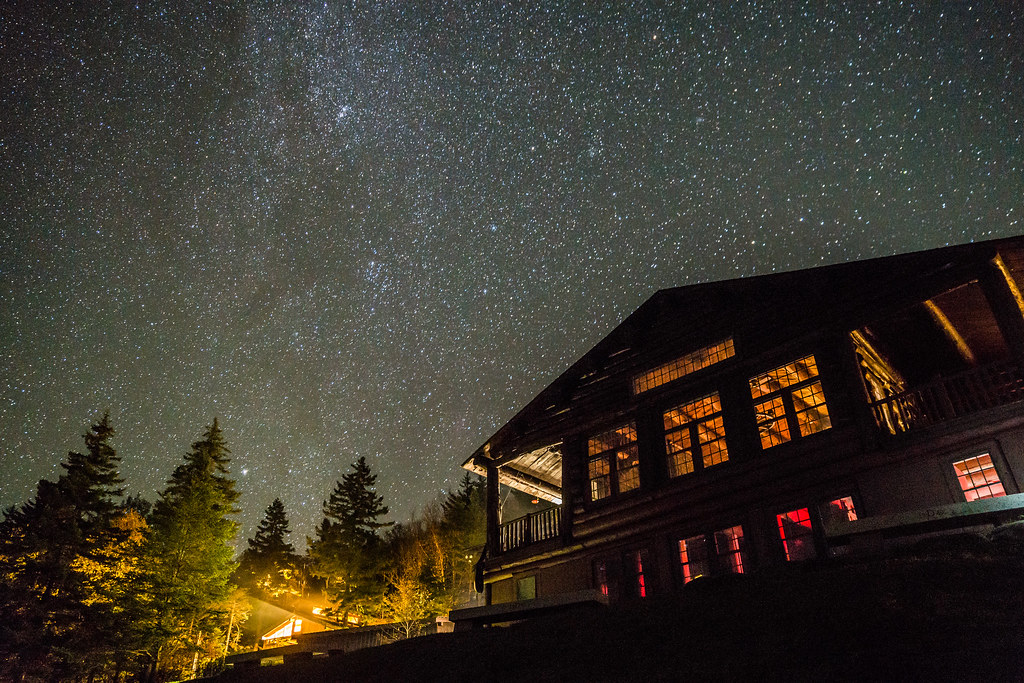The night photograph captures a serene, forested landscape under a sky brimming with stars, which almost appear unreal due to their abundance. The moon's rays illuminate the celestial expanse, hinting at the presence of possible northern lights. Below this star-studded sky is a dense forest of tall pine and aspen trees, creating a perfect backdrop for two distinct homes. On the left, a smaller house emits a welcoming glow, while on the right stands a substantial log cabin. This two-story cabin features large, uncurtained windows, a porch, and walkways. The top floor windows radiate a warm yellow-orange light, contrasting with the red glow from the ground floor. The forest and houses blend harmoniously, with the ground-level perspective giving prominence to the vast, starry sky and the encompassing natural beauty.